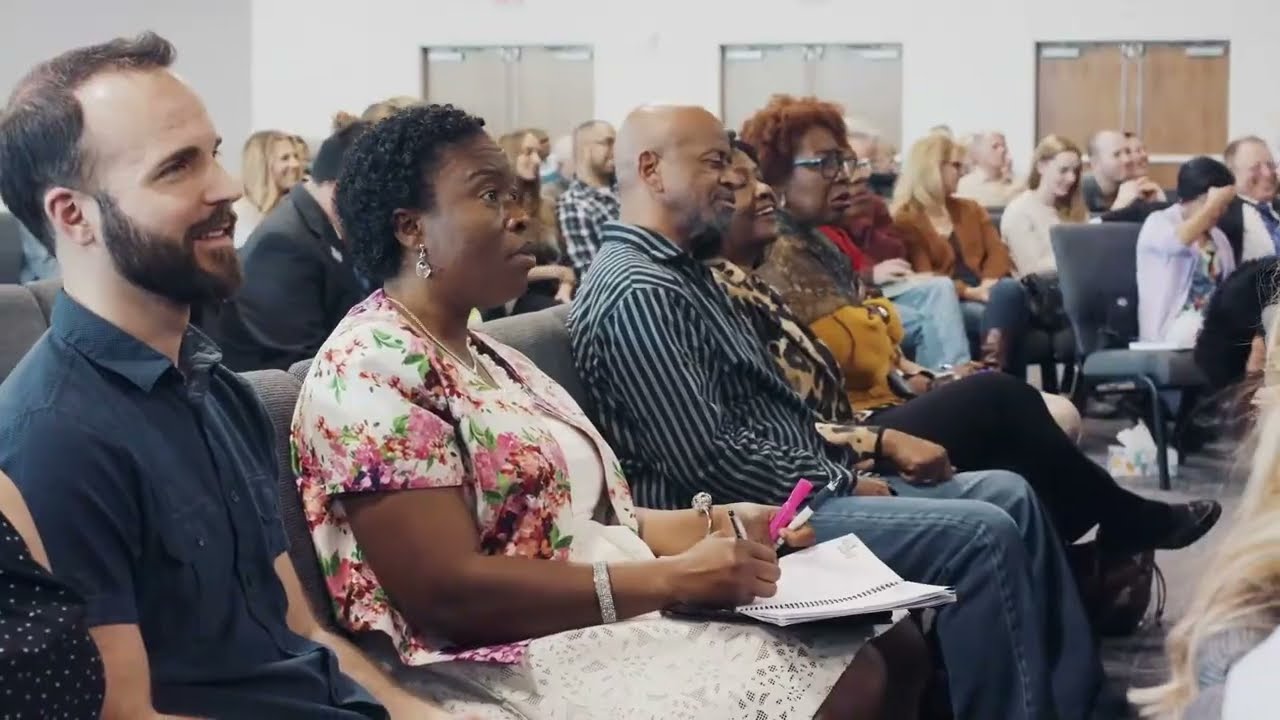This photograph captures a lively and diverse audience seated in a modestly-sized auditorium with rows of movable, cushioned gray chairs devoid of armrests. The audience appears to be engaged in a joyful event—possibly a wedding, graduation, or community meeting—given the celebratory atmosphere evidenced by the numerous smiles and laughter. People are dressed in semi-formal attire featuring button-up shirts, ties, and nice dresses yet without extreme formality such as tuxedos. The interior features white walls and a set of three pairs of gymnasium-style swinging doors in the background, indicating a multi-purpose community space. Among the attendees, a notable detail is a woman with short black curly hair in a white dress adorned with pink flowers who has a box of tissues under her seat and is raising her hand, suggesting she might be a key participant in the ongoing proceedings. Seated next to a smiling Caucasian man with a beard and mustache, she is part of a racially diverse audience, including several other people of African descent. The audience is facing the right side of the image, focusing intently on an unseen speaker or event, creating a sense of collective anticipation and enjoyment.